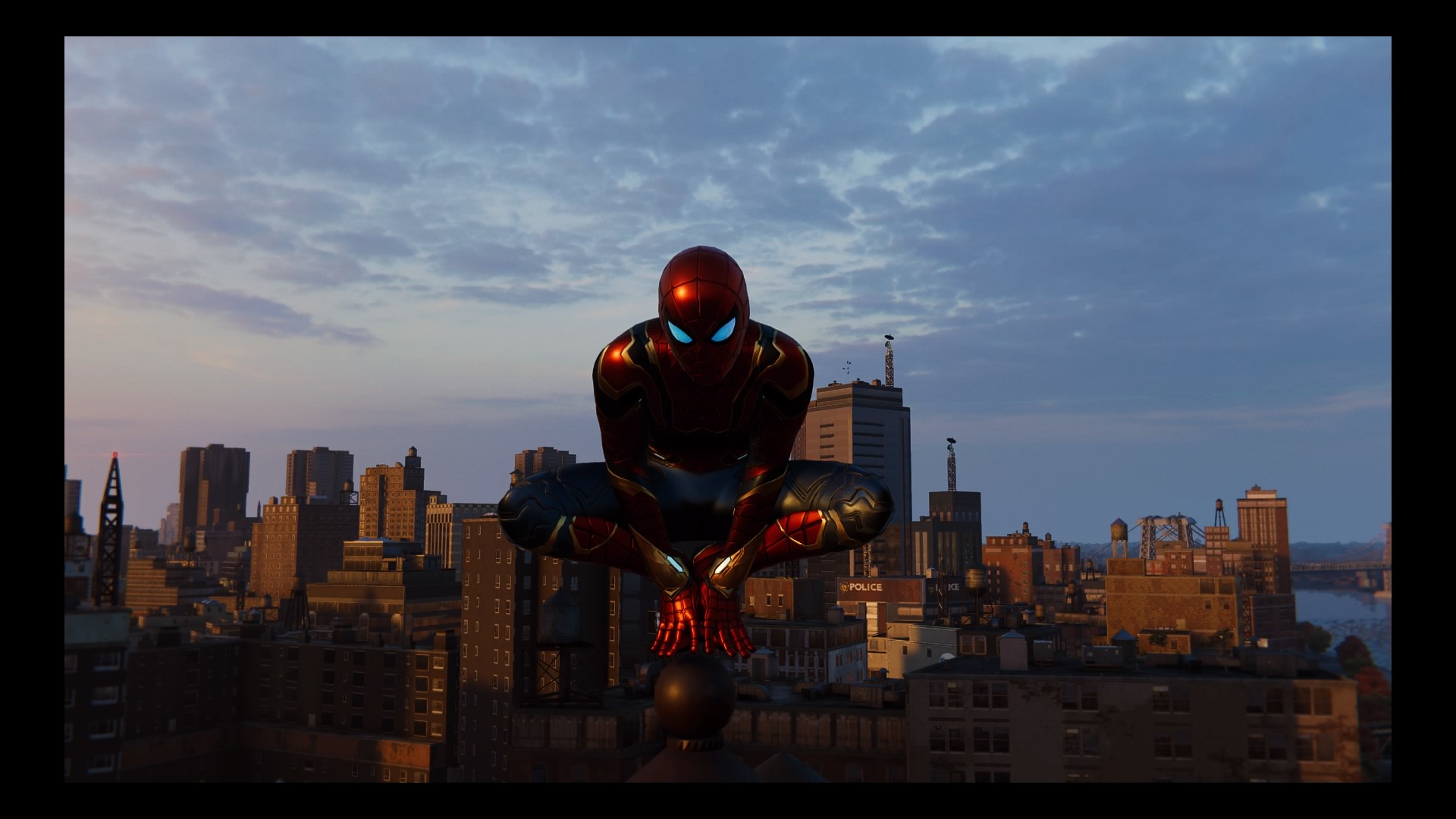The image is a detailed screenshot from a Spider-Man game, potentially depicting Spider-Man in the Iron Spider suit, which was given to him by Tony Stark in "Infinity War." It shows Spider-Man crouched atop a tall building column, overlooking a city skyline reminiscent of New York City. The sky in the background transitions from a pinkish hue on the left, likely indicative of sunrise or sunset, to a grayish-blue with clouds, suggesting an overcast day. Spider-Man's suit features a striking combination of red, black, and gold, with some parts appearing illuminated. The borders of the image are black, framing this dynamic scene.